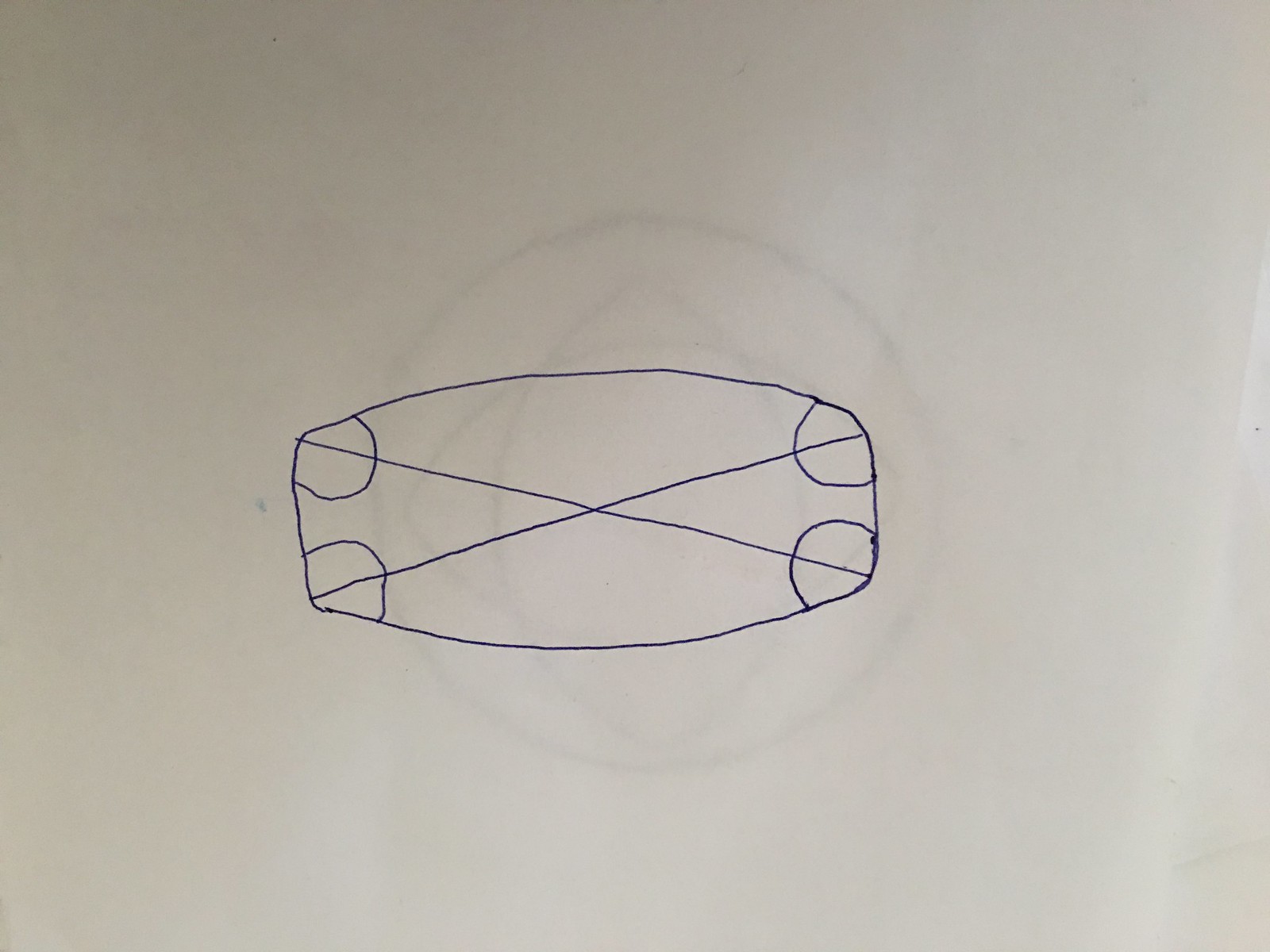On a piece of drawing paper, a faint yet discernible outline of an image from another page underneath shines through. The visible image beneath appears to be a black ink drawing of a circle, intersected horizontally and vertically by shapes that resemble an eye or rugby ball. This rough outline hints at a peculiar, abstract eyeball-like design. 

On the top sheet, there is a separate drawing done in blue biro. The primary figure is a rectangle with rounded corners, evoking the appearance of pockets on a snooker table in each corner. Within this rounded rectangle, two diagonal lines intersect, stretching from the top right corner to the bottom left, and from the top left corner to the bottom right.

This composition of overlapping images creates an intriguing and detailed visual where abstract and geometric forms blend together.